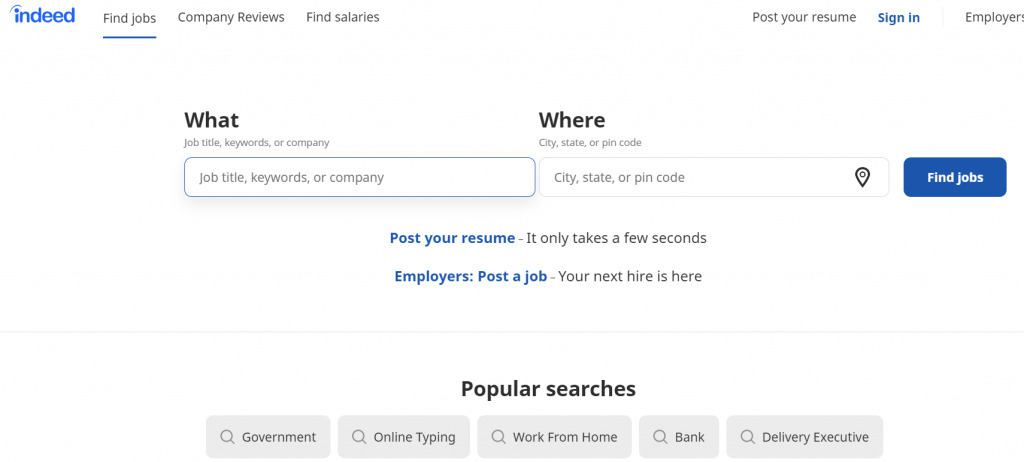The image depicts a webpage from Indeed with a predominantly white background. In the upper left corner, the recognizable Indeed logo is prominently displayed, featuring a blue, lowercase "i" with a curved line over it. To the right of the logo, the navigation bar contains several elements: "Find Jobs" in gray with a blue underline, followed by "Company Reviews" and "Find Salaries" in gray. Further to the right, the options "Post your resume" and "Sign in" are in blue, while "Employers" is in gray.

Below the navigation bar, there is a section with two input fields. On the left, the field is labeled "What" in bold, and beneath it, in smaller font, it reads "job title, keywords, or company." The input box below also displays "job title, keywords, or company." On the right, the field is labeled "Where" in bold, and beneath it, it reads "city, state, or pin code" in smaller font. The corresponding input box also shows "city, state, or pin code" and features a small location tag icon on its right side. Adjacent to this field is a blue button with "Find Jobs" written in white.

Centered below these fields, a prompt encourages users to "Post your resume" in blue, followed by a note in gray stating, "it only takes a few seconds." Further down, another centered prompt addresses employers: "Post a job" in blue, with the message "Your next hire is here" in gray. A very faint horizontal line separates these sections.

In the center of the image, the heading "Popular Searches" appears in bold. Beneath this heading are five gray boxes with slightly darker gray text and search icons. From left to right, the boxes read: "Government," "Online Typing," "Work From Home," "Bank," and "Delivery Executive."